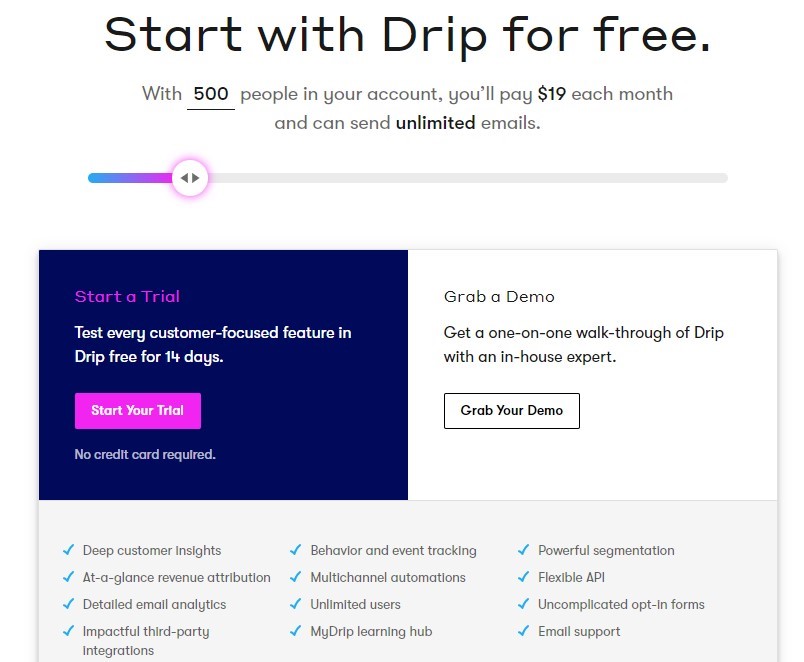"Explore the Drip platform with the free trial offer prominently displayed. Start for free, and with up to 500 contacts in your account, pay just $19 per month to send unlimited emails. The blue box invites you to 'Start a Trial' where you can test every customer-focused feature of Drip free for 14 days, no credit card required. Additionally, there's an option to schedule a personalized demo with an in-house expert for a comprehensive walkthrough of Drip's capabilities.

Below the trial offer, the site lists Drip's key features: deep customer insights, behavior and event tracking, powerful segmentation, revenue attribution, multi-channel automations, a flexible API, detailed email analytics, support for unlimited users, straightforward opt-in forms, and impactful third-party integrations. Also highlighted are the My Drip Learning Hub and email support options for users."